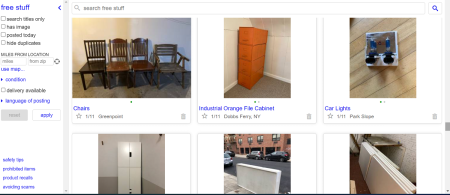In this image, we observe a screenshot from a website. The left-hand side features an array of filter options including "Free Stuff," "Search Offers Only," "Has Image," "Posted Today," and "Hide Duplicates." Below these, categories such as "Miles from Location," "Use Map," "Condition," "Delivery Available," and "Language of Posting" are displayed. Some additional buttons at the bottom left are too small to be read clearly.

At the top center, there is a prominent search bar labeled "Search Free Stuff." Beneath this search bar, six photos are displayed in two rows of three.

In the top row, the first image is labeled "Chairs" and depicts four different chairs. The second image is tagged "Industrial Orange File Cabinet," showcasing a sturdy orange file cabinet. The third image is marked "Car Lights" and displays various car light components.

In the bottom row, the titles of the three pictures are cut off. However, the first image appears to be a cabinet set and some sort of shelf. The last image in this row displays several planks of wood, neatly arranged on their sides.